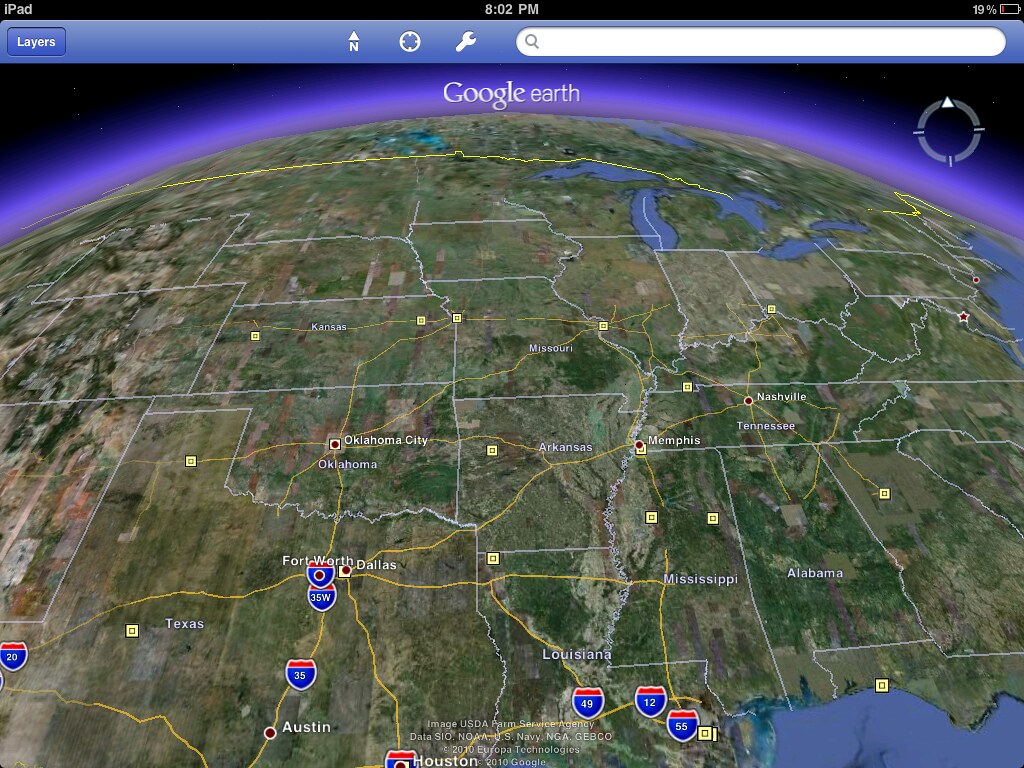This detailed Google Maps view showcases a significant portion of the continental United States, with a primary focus on Texas and Louisiana in the foreground. In addition to these southern states, the map highlights major interstates such as I-35, I-49, I-12, and I-55. Prominent cities like Dallas, Houston, and Austin are clearly marked, as well as more distant cities like Oklahoma City, Memphis, and Nashville. The map's eastern boundary doesn't extend much into the seaboard, but it does include a star denoting the capital, Washington, D.C. The visual perspective suggests an upward gaze towards the top of the earth, transitioning from a purple hue to the deep navy of space. The Great Lakes are distinctly visible, and state lines are overlaid in white, creating a clear demarcation of regions. The land areas are depicted in varied shades of greens and tans, reflecting the diverse landscape characteristics.